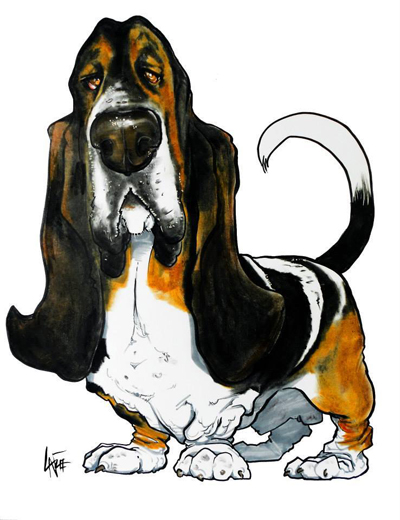This is an illustration of a basset hound on a white background, rendered in a pen and watercolor style. The overall look is very cartoony and exaggerated, with the dog having a distinctively large, shiny, wet nose and small eyes that appear tired and contemplative. The hound stands facing the viewer, appearing droopy with a comical expression. He has very long ears that turn up at the ends, reaching down near his chest, and his eyes are red with a tired, heavy-lidded look. His fur coloration is a mix of tan, black, brown, and some lighter, almost gingery tones. The basset hound's large, fat paws and overall droopy, slumped posture add to the exaggerated, funny aesthetic. The illustration is simplistic in that it has no background elements. The dog’s tail curls up towards the left, and there is a partially readable signature in the lower left corner that appears to start with the letters "L-A."